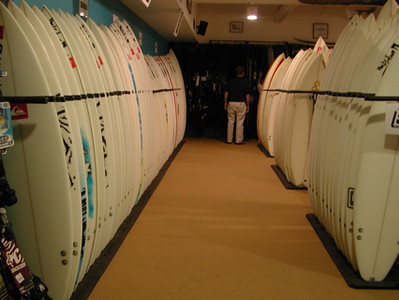The photograph depicts an indoor scene within a surfboard factory featuring a dimly lit walkway flanked by surfboards on both sides. The path, laid with a brownish surface, leads to a man standing at the far end. He is wearing a dark-colored shirt and light-colored jeans or white pants. The surfboards, mostly white and secured by black straps, display various designs with splashes of gold, red, and blue paint. A light fixture is visible on the ceiling, adding to the industrial ambiance of the space. The overall setting is somewhat dark, contributing to the factory-like atmosphere.